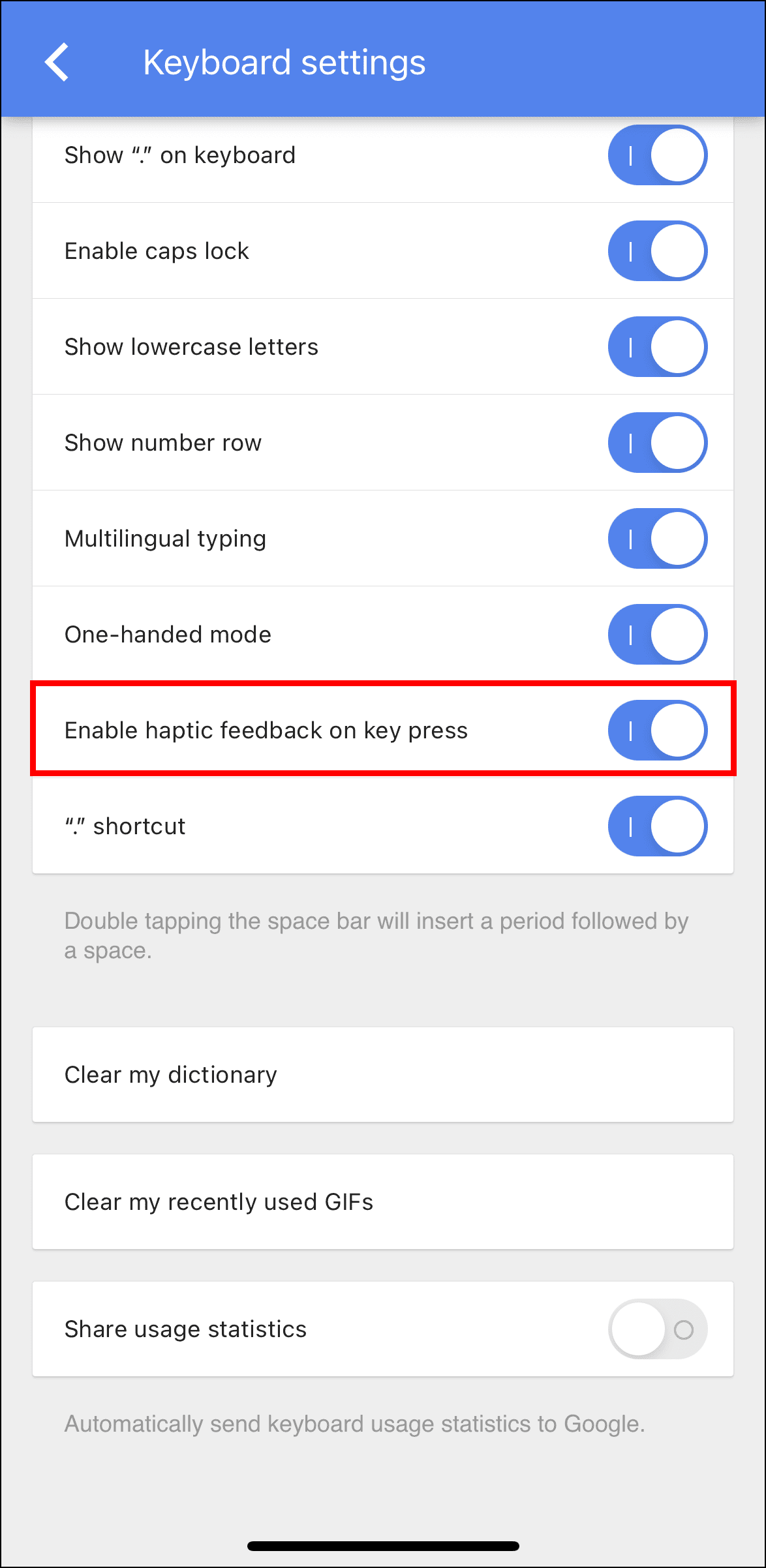A detailed screenshot of the settings page on a tablet or smartphone displays several keyboard customization options. The top bezel is dark blue with a bold white arrow pointing left and the text "Keyboard Settings" in bold white font. 

The settings include multiple sliders, each set to the right, indicating they're enabled. These sliders have blue backgrounds and white circles with a dark blue edge.

The settings listed from top to bottom are:

1. "Show '.' on keyboard" – This is displayed in black text.
2. "Enable Caps Lock"
3. "Show Lowercase Letters"
4. "Show Number Row"
5. "Multilingual Typing"
6. "One-Handed Mode"
7. The option "Enable Haptic Feedback on Keypress" is marked by a red rectangle for emphasis. "Haptic" is spelled out clearly as "H-A-P-T-I-C."
8. "'.' Shortcut" – This setting is followed by explanatory text in dark gray: "Double tapping the space bar will insert a period followed by a space."

Below these sliders, three white rectangles with black text, bordered in light gray, present additional options:

1. "Clear My Dictionary"
2. "Clear My Recently Used GIFs"
3. "Share Usage Statistics" – This includes a slider with a white circle positioned left, indicating it is off, and gray on the right side. A small black circle appears next to it.

At the bottom, gray text on a dark gray background explains, "Automatically send keyboard usage statistics to Google."

An oval navigation button is featured at the very bottom of the page.